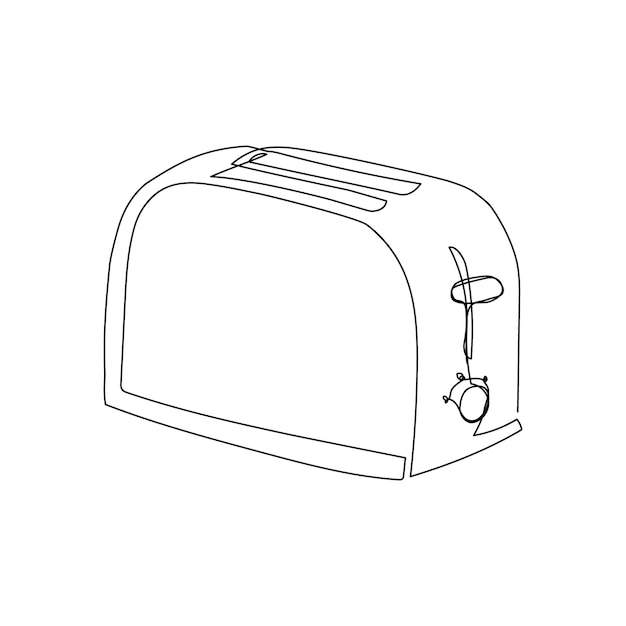The image is a minimalistic digital drawing of a two-slot toaster, rendered in simple black lines against a white background. The artwork employs a continuous line style to outline the form and shape of the toaster. Notably, the toaster features two top slots and a plainly illustrated front panel, which includes a circular knob for adjusting toasting levels and a handle bar for pushing the toaster mechanism down. The drawing is very basic and uses no colors or background elements, making it a stark and straightforward representation of a toaster.